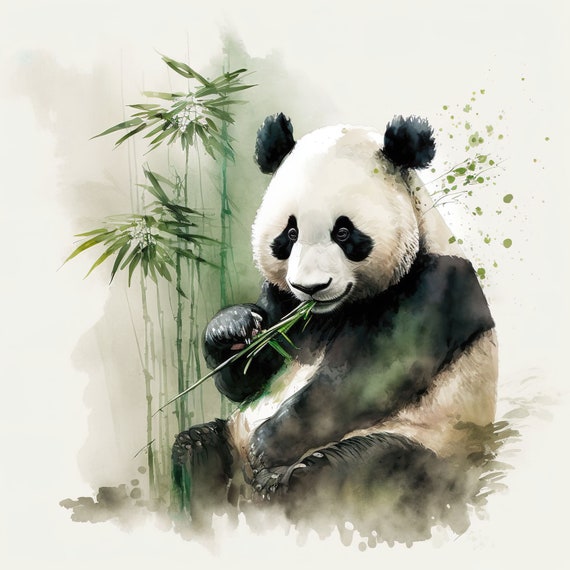This square watercolor-style painting features a large panda bear, characterized by its distinctive black and white fur—the black ears, eye patches, arms, and legs, contrasting against its white face and body. The panda is depicted in a relaxed, seated position on the ground, which is a mix of dirt and sparse grasses. The happy panda is chewing on a piece of bamboo held in its right paw, while its left paw rests casually in its lap. Surrounding the panda are several green bamboo plants with lush stems and leaves. The background is a creamy, light gray with subtle dots, suggesting an abstract or undefined backdrop. The painting has a Japanese-inspired aesthetic, with the central figure in focus against ample white space.